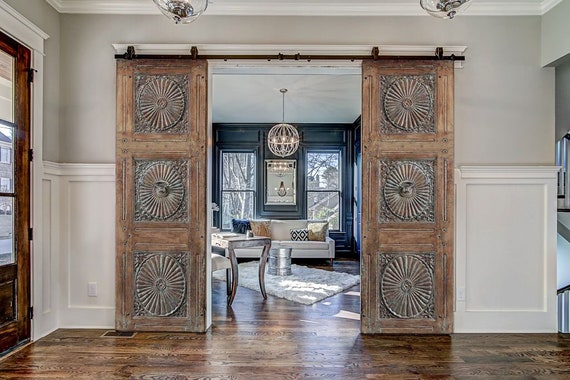The photograph depicts a meticulously designed entrance area leading into a stylish living room. The entry features elegant sliding wooden doors adorned with intricate decorations. Stepping into the living room, one is greeted with polished hardwood floors and walls painted in a dramatic dark blue. The far wall boasts large windows revealing an outdoor winter landscape with barren trees and distant views of another house, emphasizing the serene ambiance.

Dominating the ceiling is a sophisticated white metal chandelier with three lit bulbs, whose glow is further reflected in a centrally positioned mirror between the windows. Below the mirror lies a long white sofa decorated with cushions in shades of blue, gold, black, and white. A plush white rug, accompanied by two silver cylindrical coffee tables, adds a touch of luxury to the brown wooden floor.

To the left, partially visible, is a distressed white desk and chair, adding a rustic charm to the otherwise modern decor. The left side of the hallway heading further into the house features another door leading outside, while the right side opens into a stairway. The impeccably maintained wooden floors and stylish furnishings create a welcoming and cozy atmosphere, epitomizing refined interior design.